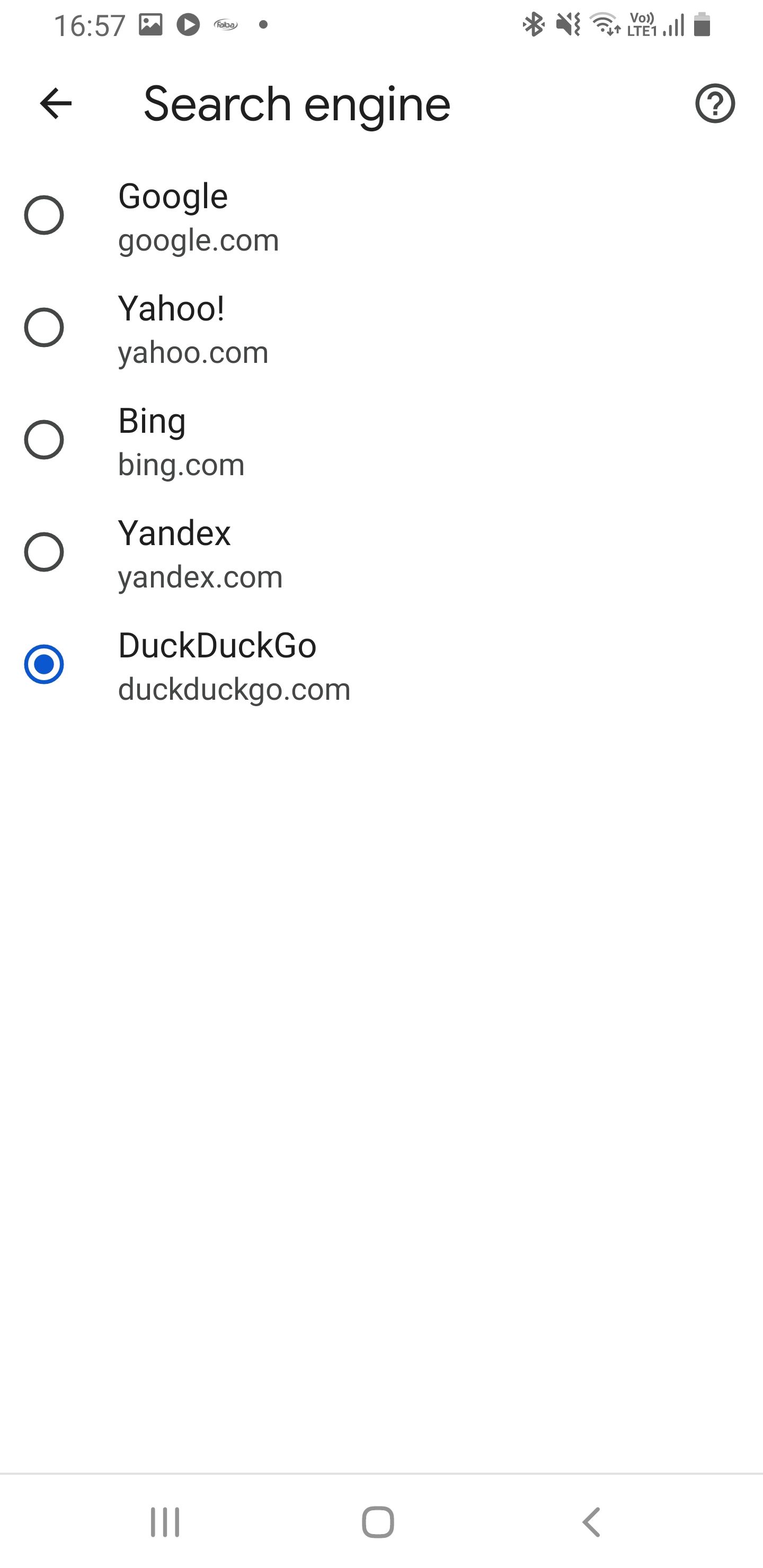The image is a screenshot from a cell phone showcasing the search engine selection and settings interface. The background is completely white, and all text is rendered in solid black. At the very top left corner, the time '16:57' is displayed. To the right of the time, there is an image icon followed by a grey dot with a white right arrow inside. Adjacent to this is some illegible text, with another grey dot positioned to its immediate right. On the far top right, there are several status indicators: a greyed-out Bluetooth symbol, a muted sound icon, Wi-Fi connectivity indicator showing 'LTE' and full signal strength with four bars, and an almost fully charged battery icon.

The main interface focuses on the search engine selection settings. At the top center of this section, 'Search Engine' is prominently displayed in large black letters. On the right side, there's a circle containing a black question mark, presumably for help or more information. Below, a list of search engine options is presented, each with a radio button to its left. The options are:

1. Google (google.com)
2. Yahoo (yahoo.com)
3. Bing (bing.com)
4. Yandex (yandex.com)
5. DuckDuckGo (duckduckgo.com)

The radio button next to DuckDuckGo is filled in blue, indicating that it is the currently selected search engine.